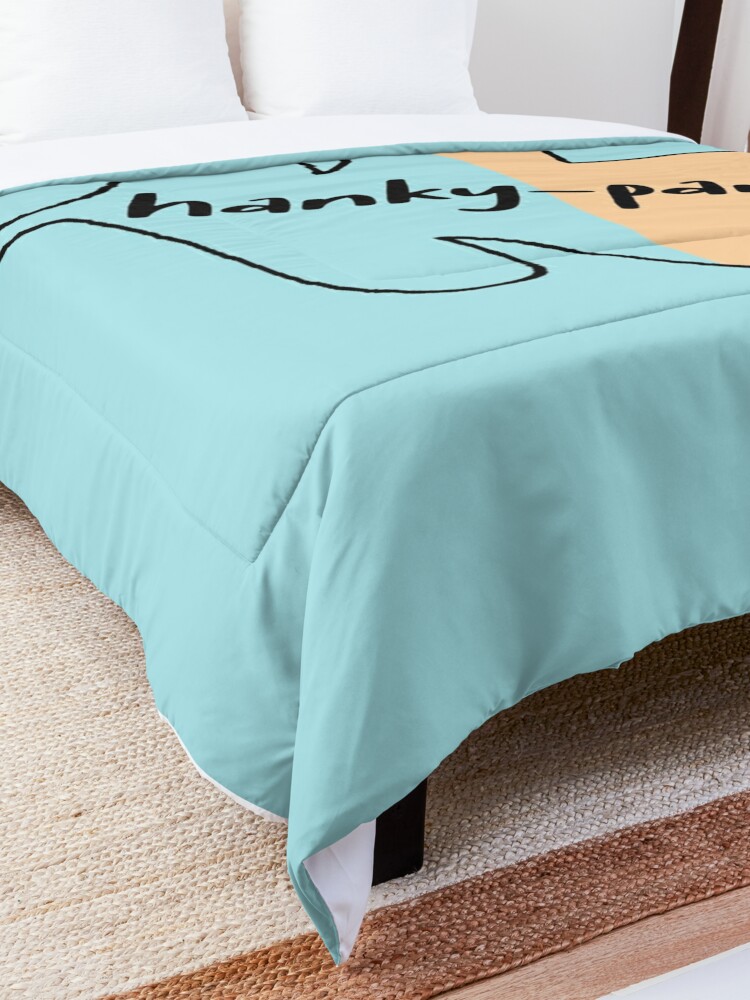This photograph captures a neatly made bed with a teal, or mint green, blanket draped over it, partially folded back to reveal a white underside. The blanket prominently features the text "Hanky Panky" in black lettering, though only "Panky" and part of "P" are fully visible due to the fold. Two white pillows rest at the headboard. A single black leg of the bed frame is visible, poking out from underneath the blanket. The bed stands on an area rug that is primarily beige, accented with a brown border. The image suggests a clean and simple aesthetic, similar to what you might find in a short-term rental listing.